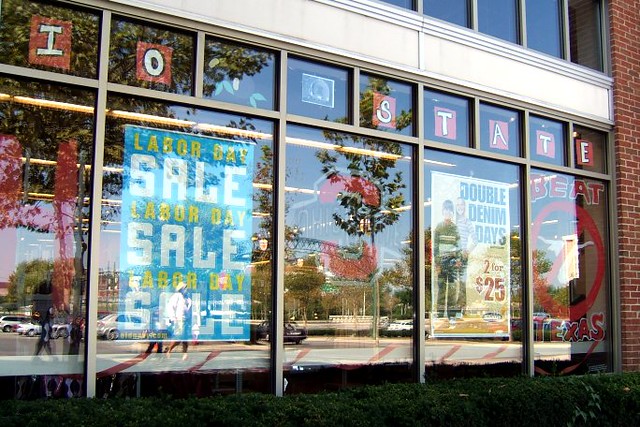This photograph captures the exterior of a store with large, glass divided windows. Prominent on one set of windows is a series of signs inside, featuring "Labor Day Sale" repeated three times. Another colorful poster announces "Double Denim Days 2 for $25" and includes an image of a boy and a girl. Painted directly on the glass, there is partially visible text saying "I-O State," likely "Ohio State," rendered in white, red, and black paint. Another set of painted text reads "Beat Texas" alongside a red circle with a slash through it, likely depicting a bull's face to symbolize the "No Texas" sentiment. At the bottom of the windows, green shrubs are visible, while reflections of the outside parking lot can be seen on the glass.